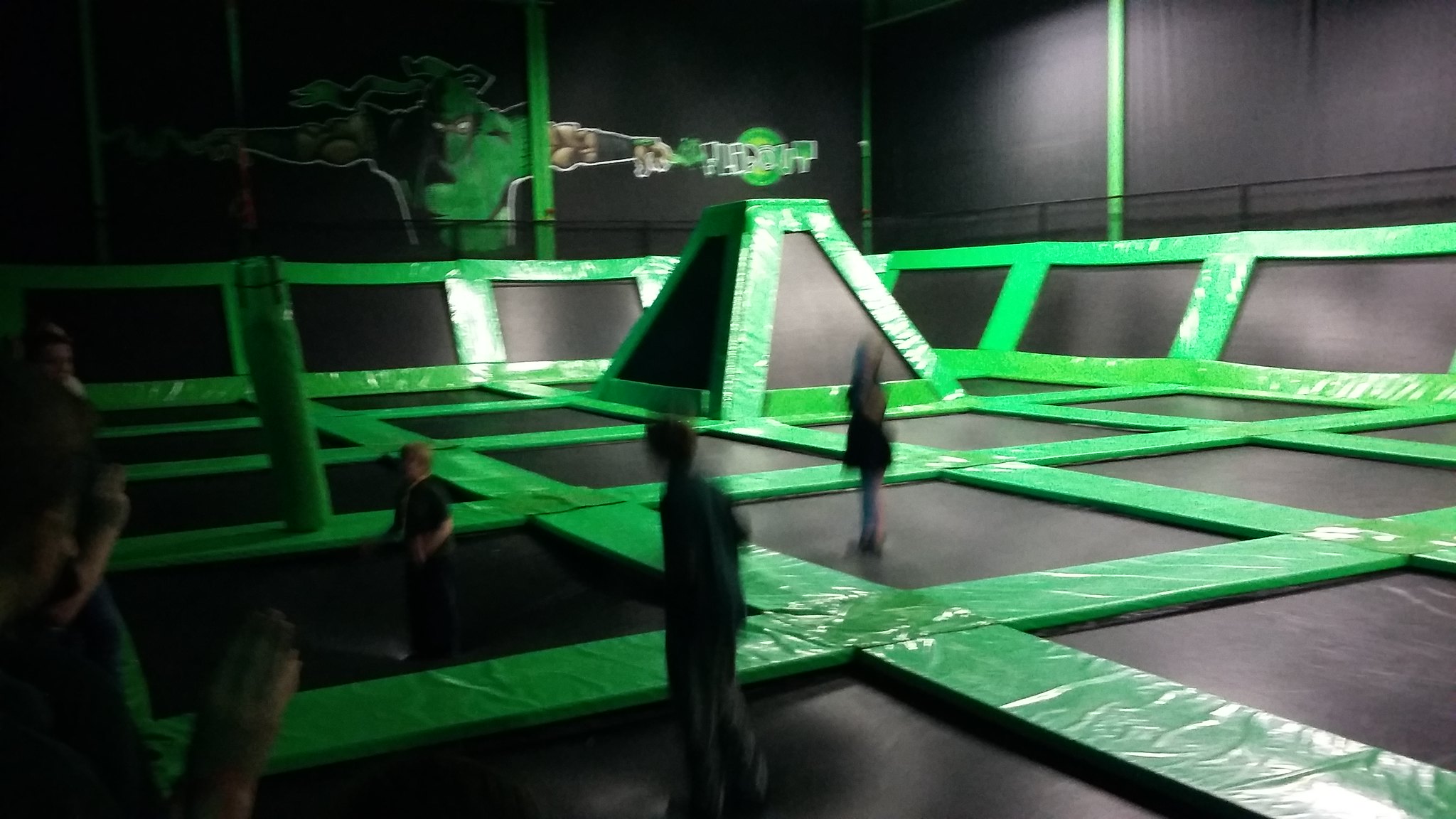The image depicts a trampoline park featuring a series of interconnected black trampolines outlined with bright green, cushioned walkways, creating a grid-like pattern. Each trampoline section is bordered with vibrant green dividers, forming a visually distinct layout of rectangular bounce areas. Towards the back of the space, there is a triangular bounce wall designed for jumping and rebounding. Above the trampolines, a black fence and matching curtains hang against the wall. On one wall, a large diagram of a green and black Marvel character, complete with bright eyes and extended arms, adds a decorative touch, though its accompanying text is indistinguishable due to the blur. The image includes blurred figures of people jumping on the trampolines, with a particularly noticeable indentation on one trampoline from the impact. On the left side, blurry spectators can be seen watching the activity, further emphasizing the lively environment.